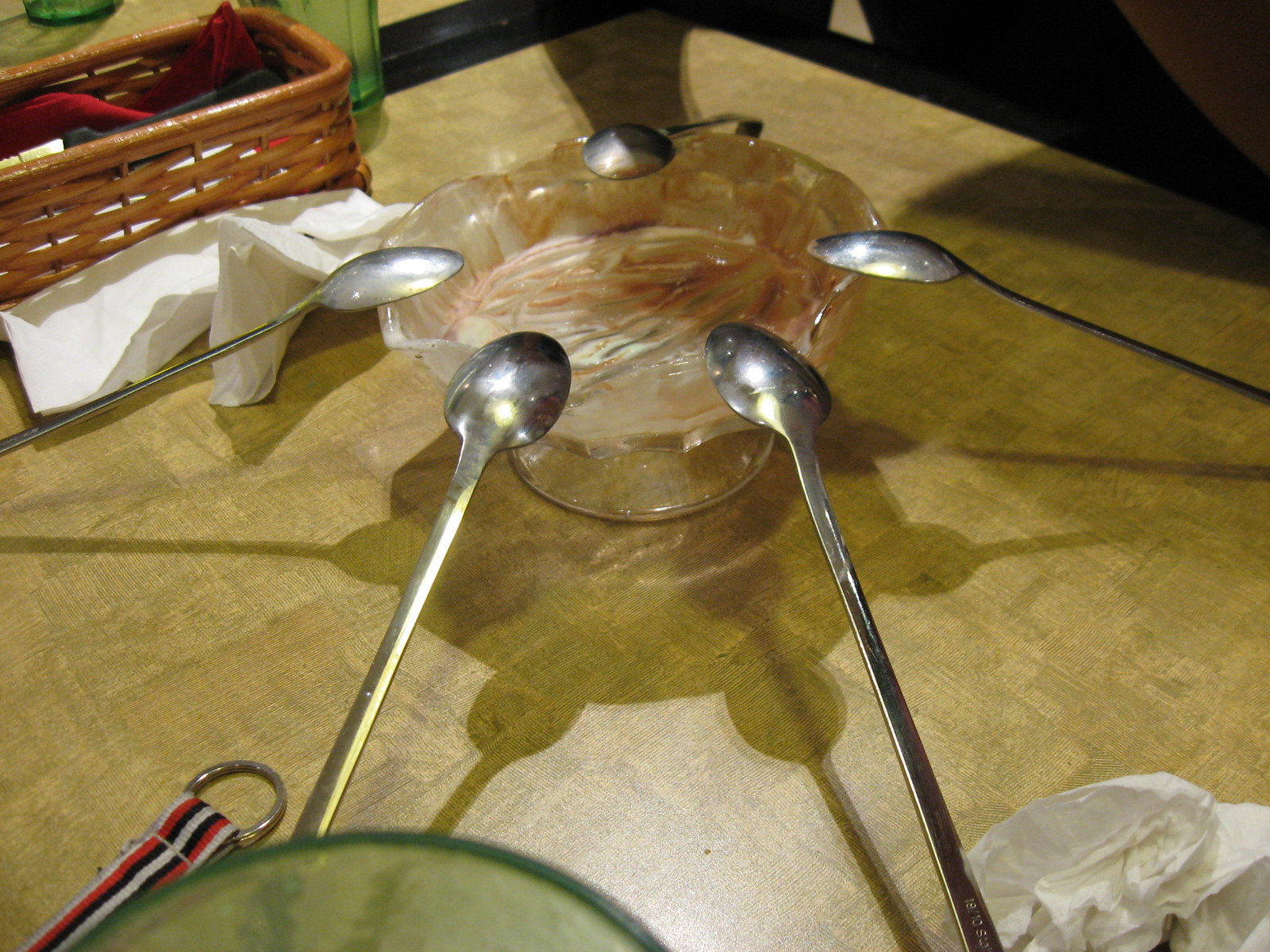The image captures a detailed scene centered around a large, scalloped glass dish on a pedestal, resembling a bowl for serving sundaes. The dish features streaks of white and brown, suggesting remnants of ice cream with chocolate sauce. Resting on the edge of the dish are five to six long-handled silver spoons, placed bowl side down, akin to those used for stirring iced tea. The setup is on a tabletop with a mixed hue of brown, green, and gold, reminiscent of surfaces found in older campers. Surrounding the glass bowl are crumpled white napkins—two prominently visible in the top-left and bottom-right corners. Additionally, a green glass bowl and a green Tupperware lid are present, along with a striped keychain or nylon strap with a hook or loop on the end. Completing the scene is a wicker basket filled with miscellaneous items, including something pink, situated in the upper left of the image. A shadow from an unidentified object casts a shape on the table, adding depth to the composition.